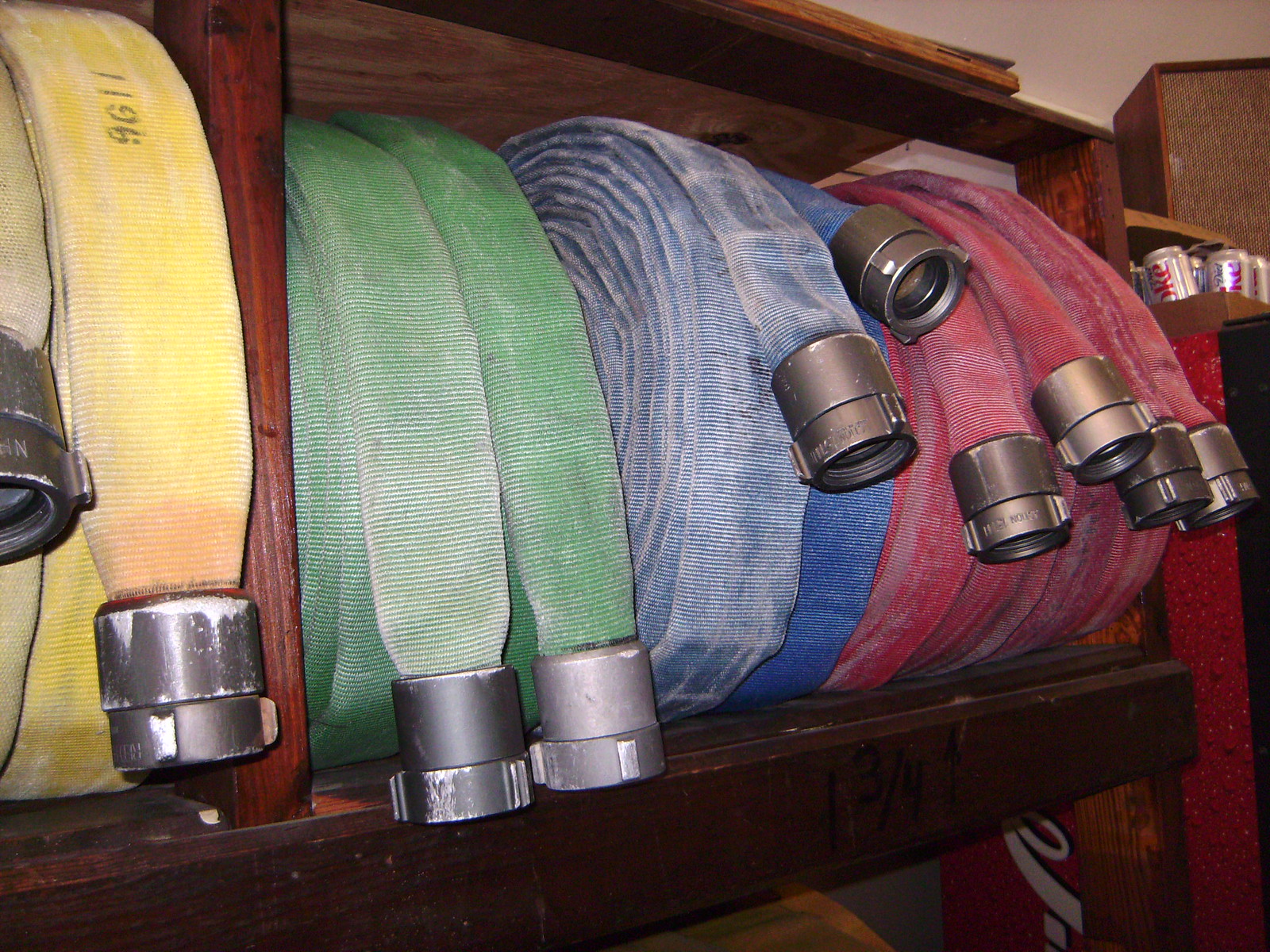The photograph displays a collection of hoses neatly arranged on a dark cherry wood shelf, seemingly expandable fabric types given their flat, tightly coiled appearance. From left to right, there are pairs of hoses grouped by color: two bright yellow hoses on the left partially cut off by the photo’s angle, positioned next to a shelf pole; next are two green hoses with the left one appearing faded and paler in color; following them are two blue hoses where the left is light blue and the right is a darker blue. Finally, there are four uniformly shaded dusty red hoses. The hoses are primarily oriented downwards and arranged in thick, numerous rolls, suggesting they are lengthy. The scene is framed with a bright red Coca-Cola vending machine on the right side, featuring the brand’s logo and water droplet design, with a brown box of Coke cans seen on top of the machine.